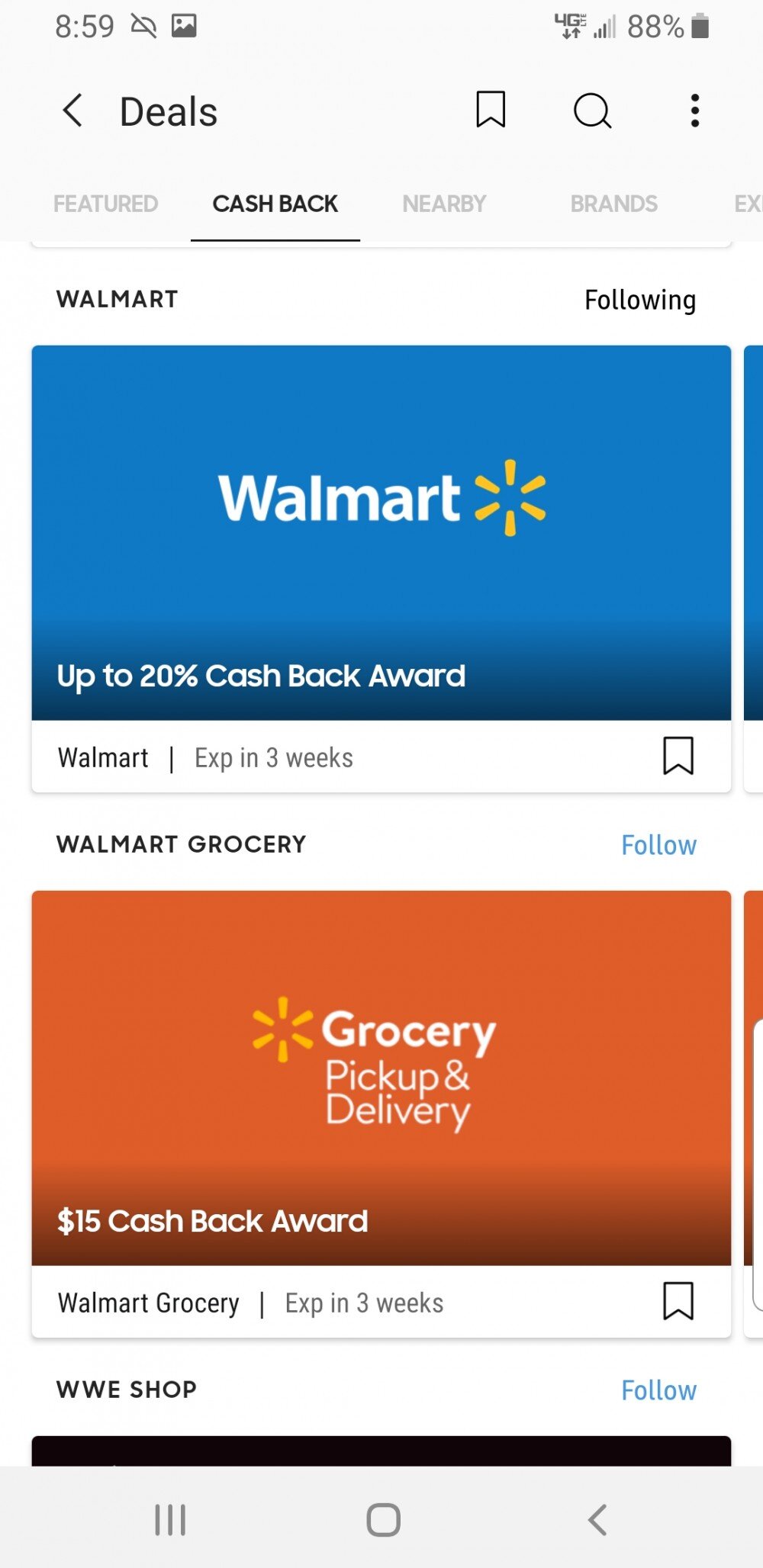This is a screenshot from a tablet or smartphone, displayed in military time with "8:59" in black text on a light gray background. A half-crescent moon icon, crossed out with a line, suggests a do-not-disturb mode. 

Adjacent to the time display, a square icon features a black circle over white, with black mountain-like shapes. To the right, a "4G" symbol with bidirectional arrows indicates data transfer status, followed by an 'E' that signifies the type of network. The signal strength shows three out of five bars, and the battery life is indicated at 88% with a corresponding icon.

Navigational icons include a black arrow next to the word "deals," a bookmark symbol, a magnifying glass icon, and three vertical black ellipses. The interface shows multiple tabs: the first tab is gray, while the selected tab, labeled "cashback" in bold black text with an underline, is active. Nearby tabs labeled "nearby brands" and a partially visible "EX" are in a faded mid-gray.

In a new white section, the bold black label "Walmart" appears, followed by the status "following" on the right. Inside this section, a dark blue rectangle displays "Walmart" in bold white text. A sun-like icon with six yellow rays resembling a gear is also present. Below, text in bold white announces "Up to 20% cashback reward." Adjacent are two rectangles—a small white one and a partially visible dark blue one, partially cut off.

Underneath, inside the white rectangle, "Walmart" appears in regular black text followed by a line, then in thin black text, "EXP in 3 weeks" and a bookmark icon. Further down, "Walmart grocery" in bold black is paired with a hyperlink "follow" in blue on the right. Nearby, a dark orange rectangle next to a partially visible one repeats the sun icon, with bold white text saying "grocery" followed by "pickup and delivery" in regular white text, and another bold white line stating "$15 cashback reward."

Subsequently, another section inside a white rectangle marks "Walmart grocery" in regular black text, the line, "EXP in 3 weeks" in thin black text, and a bookmark icon underneath. 

Right after, "WWE shop" in bold black text is paired with a blue hyperlink "follow." Finally, a black rectangle band is overlapped by a mid-gray rectangle housing three black lines, a black circle, and a black arrow.